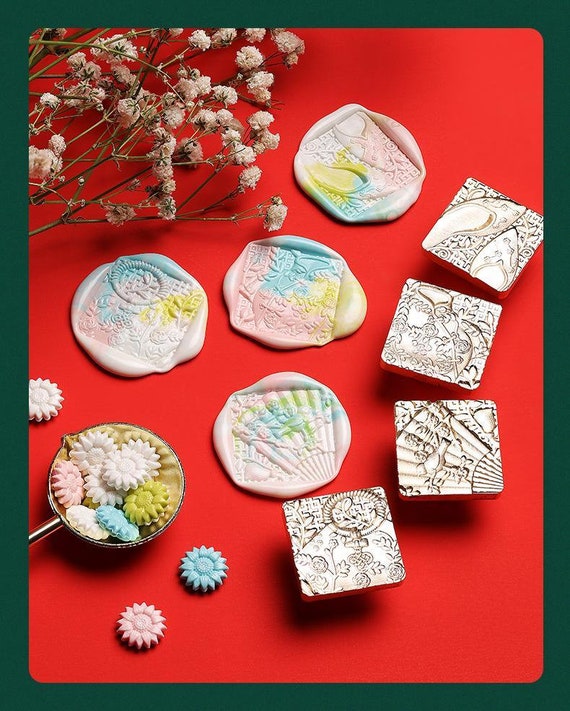The image features a detailed and carefully arranged setup of home decor or bath objects, viewed from a bird's eye perspective. Centered on a vivid red background, the arrangement includes multiple pastel-colored items such as blues, pinks, yellows, and whites. Prominently displayed are four to five pieces resembling soap or stamped wax seals, each featuring intricate oriental or floral bas-relief designs. At the top, the composition is complemented with dried flowers for added decorative flair. Below these central items, a small dish holds numerous flower-shaped soaps or wax melts. To the right are four distinct, floating stamp-like tools, possibly for creating the detailed imprints seen on the soaps or wax pieces—suggesting that the entire setup might indeed be computer-generated. The overall setting appears to be an indoor scene meticulously laid out to showcase the aesthetic and functional aspects of these decorative or bath items.